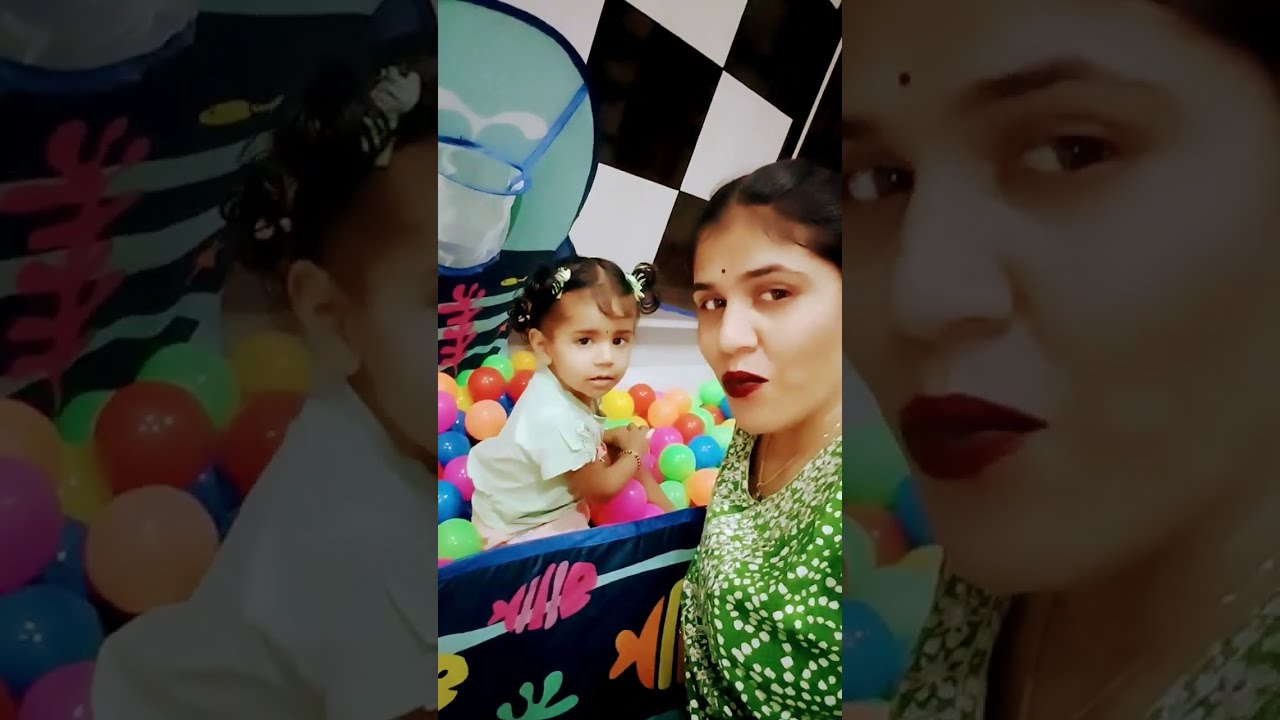The image depicts an indoor play area centering around a woman and her young daughter. The scene is split into three columns, with the left and right columns significantly tinted. In the right column, through the tint, a close-up reveals the woman's face. She has dark red lips, a red dot on her forehead, and her eyes are slightly turned to the right while her face is tilted to the left. Her complexion is olive, and she appears to be of Indian descent.

The clear middle section reveals more detail: The woman wears a green shirt adorned with white dots and has black hair. She stands beside her young daughter, who is playing in a ball pit. The child, with black hair styled in ponytails parted in the center and some bangs falling on her forehead, wears a very light green shirt that reaches just above her elbows. The ball pit is filled with balls of various colors, including red, peach, purple, blue, and green. The ball pit has a mostly black border with a blue top edge featuring a white stripe and colorful fish illustrations, prominently showing a pink fish.

The background of the central section features a black and white checkerboard pattern, adding contrast to the scene. Additionally, there is an image of a glass with a red straw in the upper left corner of the middle section. The left column presents a close-up of the back of the child's head, where her ear is visible, captured through another tinted filter.